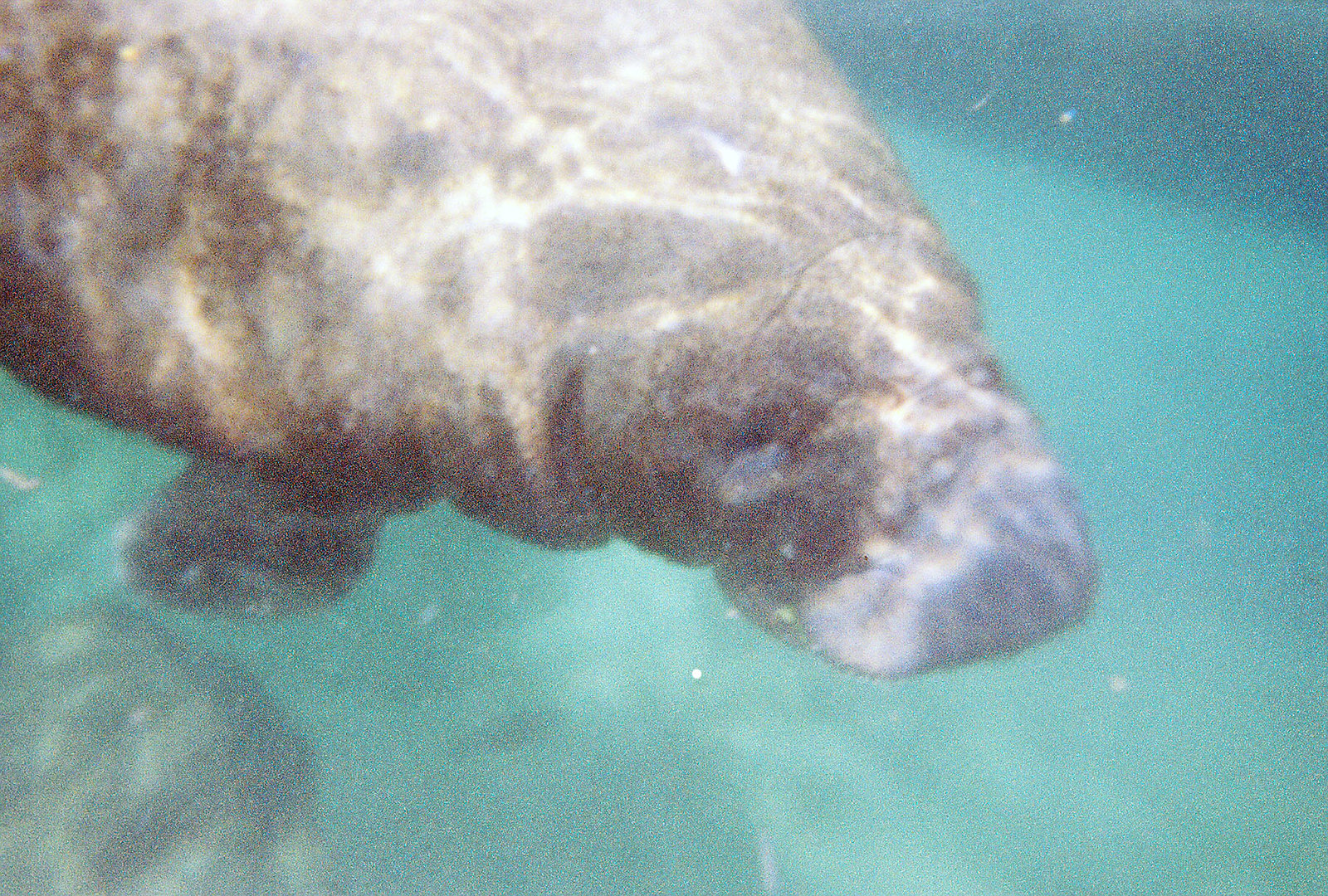The photograph captures a large, brown manatee swimming in clear, lightly tinged greenish-blue water, likely within a pool or water reservoir such as those found in aquariums, water parks, or zoos. The photo, rectangular and faded in quality, suggests an older, possibly scanned physical image, adding a grainy texture. The manatee's body stretches from the upper left corner, with its face descending close to the lower right corner. Sunlight refracts through the clear water, creating highlights on the manatee's back. Although the manatee's face is quite blurry, its body, with varying shades of brown and one visible flipper, contrasts against the sand-colored bottom. There may also be the hint of another manatee in the lower left-hand corner of the image.